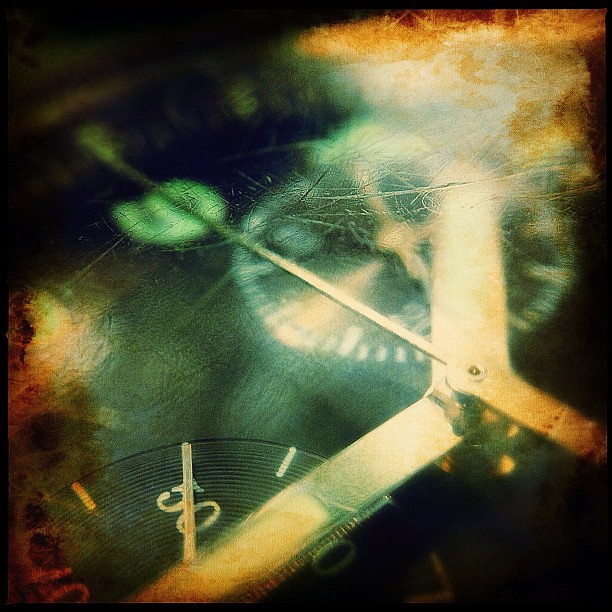This artistic color photograph is a close-up of an analog clock or possibly a watch, set against a black background with splashes of light. The main dial, which appears green with tinges of gold, dominates the composition. A prominent silver hour hand extends diagonally from the top right light source, rich with an orange outer glow, down toward the bottom right. A slender sweep second hand also moves across this surface, catching the light. The clock face features regular numerical markings, including visible digits like 9, 10, 20, 40, and 50. Additionally, there is a smaller white clock face situated toward the upper left under the light source, marked with white digits and hands.

The glass covering the main clock face is deeply scratched and unevenly discolored with a splotchy brown substance, hinting at a history of use and age. A partially visible secondary clock face at the bottom left, with a smaller white hand on the 50, adds to the complexity of timekeeping elements in the image. The intricate interplay of light and shadows, along with the detailed textures of the clock, create a striking and evocative visual narrative.